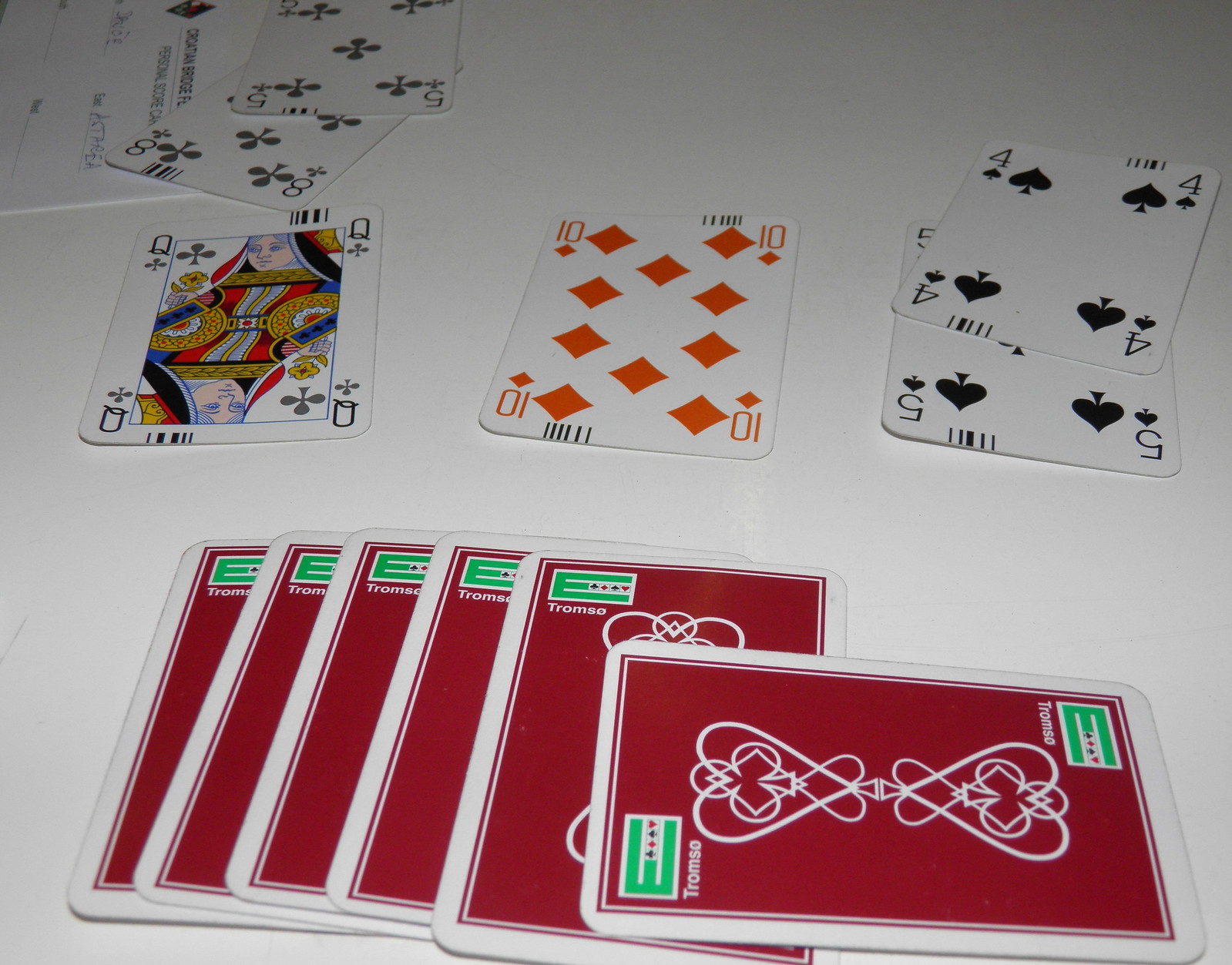This image captures an engaging game of cards in progress on a pristine white table. Several cards are prominently displayed face-up, including the Queen of Clubs, the Ten of Diamonds, the Four of Spades, the Five of Spades, the Five of Clubs, and the Eight of Clubs. The black suits of Clubs and Spades contrast strikingly with the red Diamonds.

Additionally, several cards are positioned face-down closest to the camera, characterized by red backs adorned with intricate, royal-themed designs featuring a club, a heart, a spade, and a diamond, all superimposed and mirrored. In two diagonal corners of these card backs, there are green rectangles, each inscribed with the word "TROMSO," accompanied by symbols of each suit: the Diamond, Heart, Spade, and Club.

In the background, partially obscured by the Five and Eight of Clubs, a white piece of paper with black text—possibly a calendar or some paperwork—adds a touch of everyday realism to the setting.